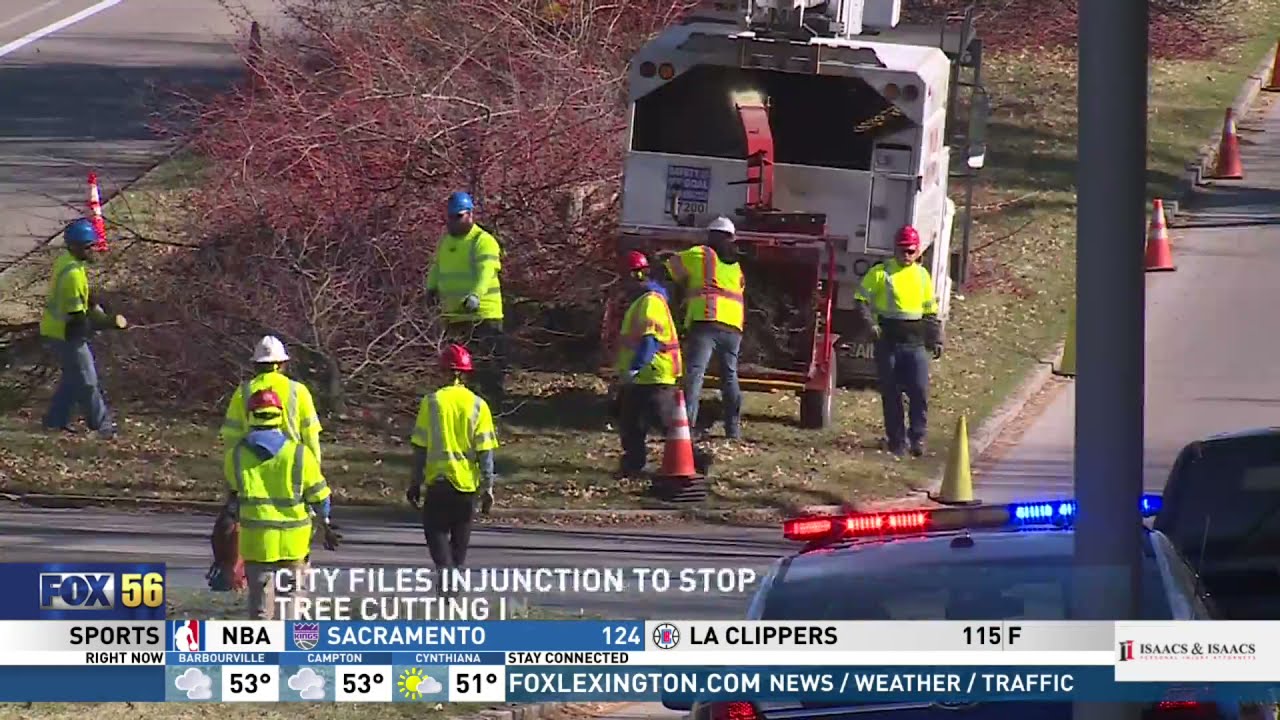This image is a detailed screenshot of a Fox 56 news broadcast showing a headline "City Files Injunction to Stop Tree Cutting". The scene features a group of eight construction workers, all wearing high-visibility yellow vests and various colored helmets—blue, red, and white—gathered around a white pickup truck and a large collection of downed tree branches. The workers are positioned in a median on a wide road, bordered by safety cones, with some bright green grass patches visible under the branches. They appear to be using a wood chipper to process the tree materials, visible with a red arm stretching into a square-shaped vehicle in the background. On the bottom right of the image, there is a cop car with flashing red and blue lights. The lower part of the screen includes information typical of a news ticker: Fox 56 branding, the headline about the tree cutting injunction, sports scores showing Sacramento 124 vs. LA Clippers 115 (final), weather information indicating 53 degrees in Barberville and Campton, and 51 degrees in Cynthiana. Additionally, it shows a URL, foxlexington.com, linking to news, weather, and traffic updates.